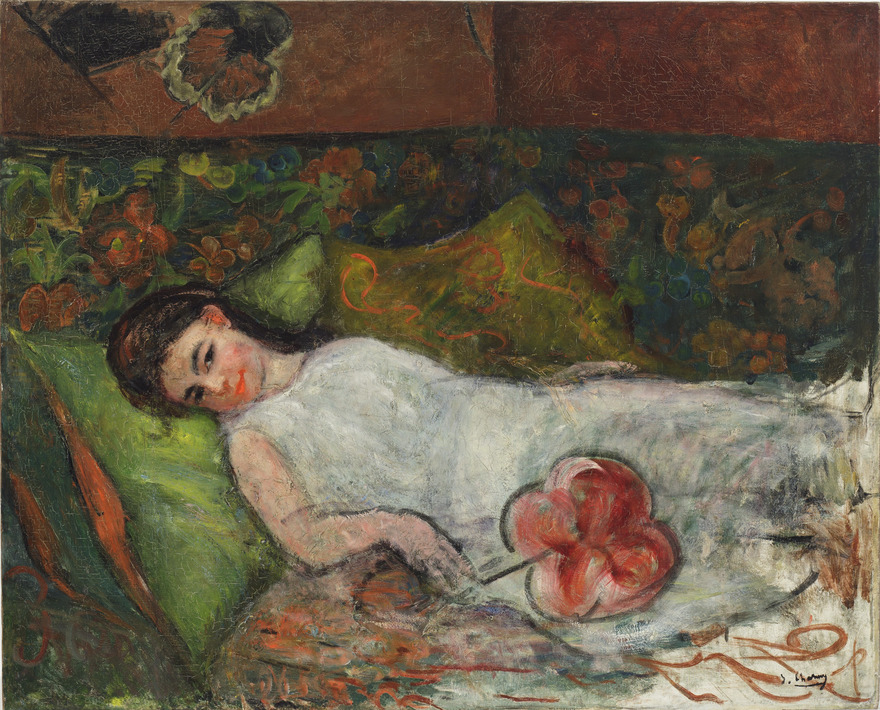This is a wide, rectangular painting depicting a girl lying down on several bright green pillows with orange borders. She is positioned with her head towards the left middle side of the painting, lying horizontally on her back, and gazing sideways, possibly towards the painter. She has dark brown hair, pale skin, and orange lips, smiling slightly. The girl wears a long, flowing white dress adorned with numerous brushstrokes in white, black, blue, red, and orange, giving it a vibrant and textured appearance. Her bent arm rests beside her, holding what appears to be a thick, red, butterfly-shaped fan or a flower with an intricate design. 

Behind her, the headboard of the couch or bed features an intricate green floral pattern. The wall above is a burnt orange color, suggesting a warm, somewhat earthy environment. The painting is notable for its wild, bold brushstrokes, giving it an almost two-dimensional appearance with a black outline around the subject. The entire scene is composed with a vivid color scheme of green, orange, yellow, turquoise blue, and brown. The bottom right-hand corner contains the artist’s signature, "Jay Lindsay," underscored by a black line.